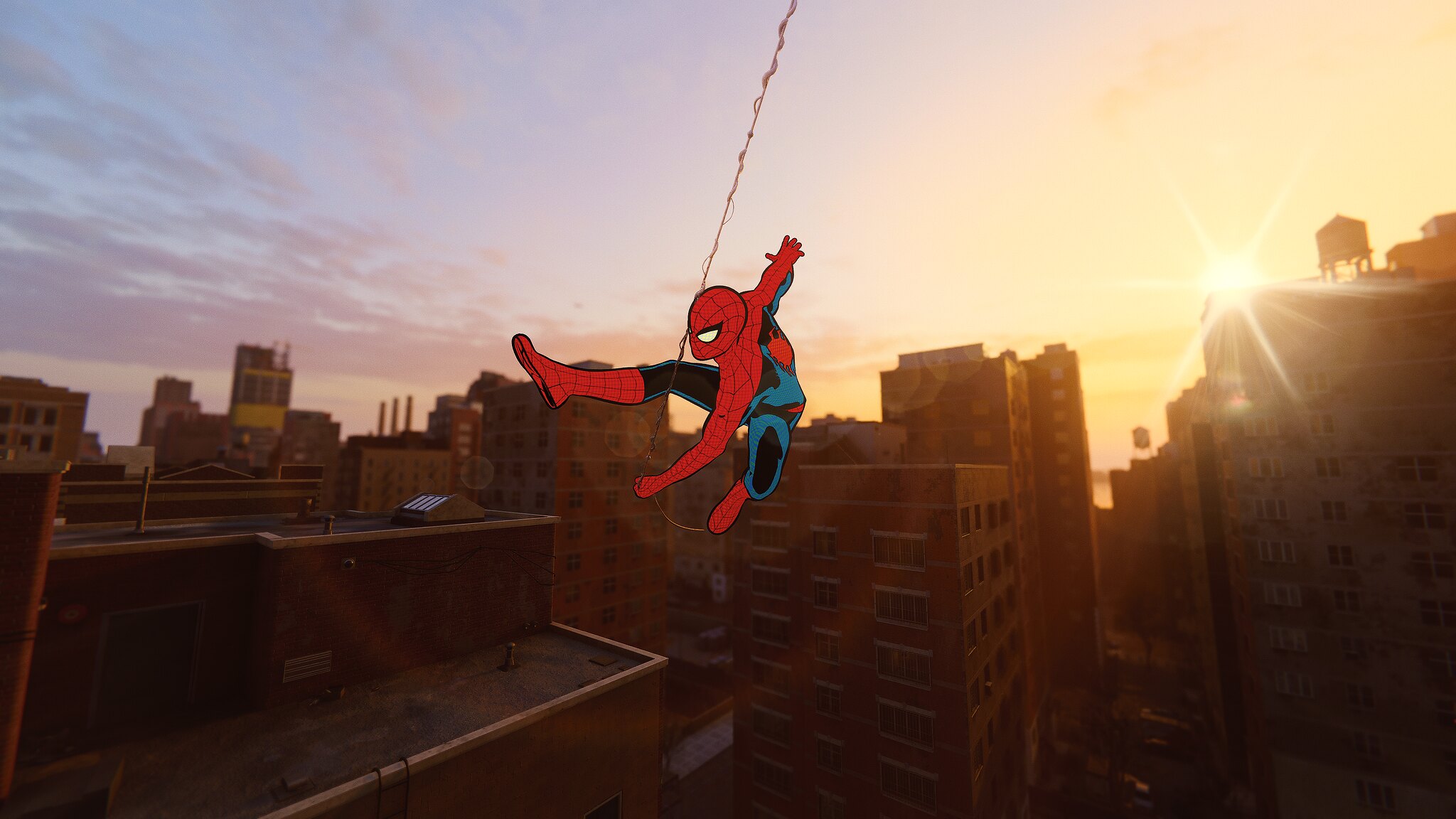This captivating photograph captures the bustling cityscape at sunset, with towering skyscrapers dominating the background. The sun is setting behind the corner of a skyscraper in the upper right, casting a warm orange glow across the sky to the right, while the left side of the scene retains the cool hues of a blue sky adorned with fair-weather clouds. In the center of the image, a dynamic cartoon figure of Spiderman is superimposed. He is in mid-flight, his left hand shooting a web that stretches from the top middle of the photograph down to the center. Spiderman’s right leg is fully extended straight, and his left leg is bent underneath him, displaying an acrobatic posture. His right arm is extended behind him as he soars gracefully over a building, adding a thrilling sense of action to the serene urban sunset.